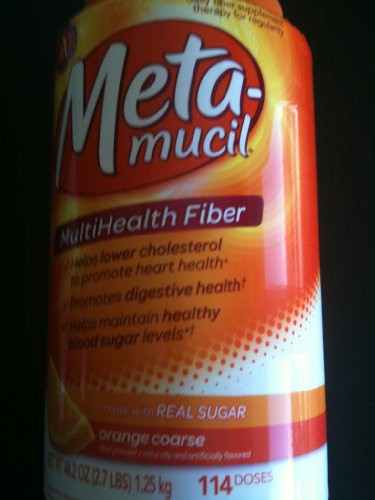A detailed caption for the Metamucil jar image could be:

"A jar of Metamucil stands out with a prominent red circle on the front, displaying the brand name in large white letters. The top right corner features text that mentions its therapeutic benefits, surrounded by a vibrant yellow backdrop with orange edges. Below, a bold red rectangle houses white text that highlights its multi-benefit fiber content, emphasizing its role in lowering cholesterol, promoting heart health, aiding digestive health, and maintaining healthy blood sugar levels. Another orange rectangle below states that the product is made with real sugar. The lower portion of the jar is decorated with an array of orange dots against a gradient background, leading to a clean white base. At the very bottom, the weight information is displayed as 2 oz (2.7 lbs, or 1.25 kilograms), and it also mentions the product contains 14 doses."